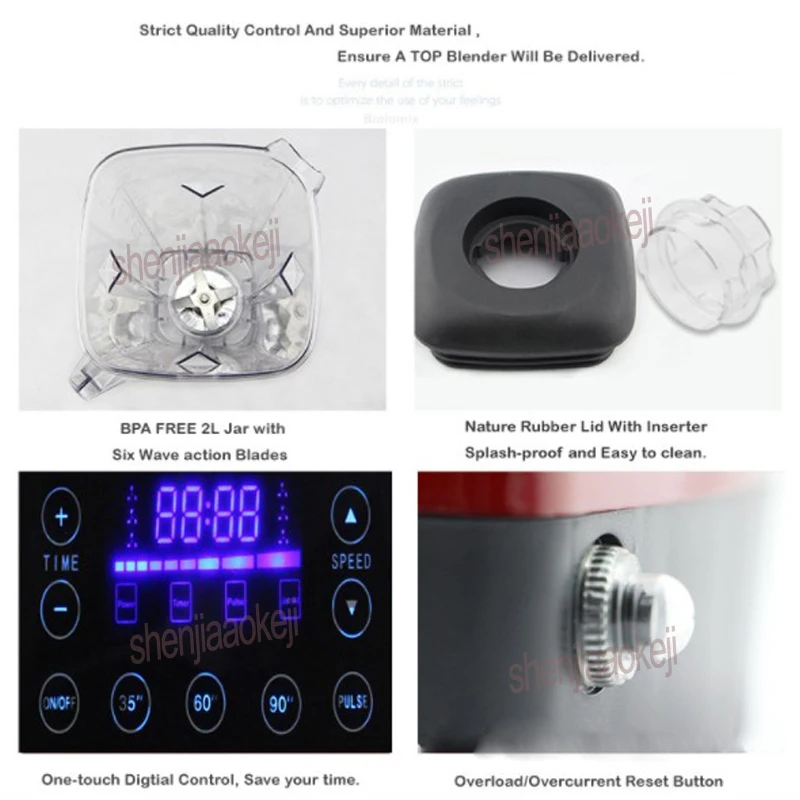The image is a detailed diagram of a blender, meticulously divided into four square photos arranged in a larger square, each illustrating different components of the appliance. The top left photo features a clear jar, highlighting the internal silver blades with a label beneath that reads, "BPA-free 2L jar with six wave action blades." To the right, the top right photo displays a black plastic square lid with a small hole in the center, accompanied by a plastic inserter piece. The text below this image states, "Nature rubber lid with inserter, splash proof, and easy to clean." In the bottom left corner, a digital control panel is shown, complete with on/off buttons and a timer, captioned, "One-touch digital control saves your time." The final photo in the bottom right shows a close-up of a knob, labeled, "Overload overcurrent reset button." The arrangement is underscored by a theme of strict quality control and superior materials, ensuring the viewer comprehends the high standards and functionality of the blender.